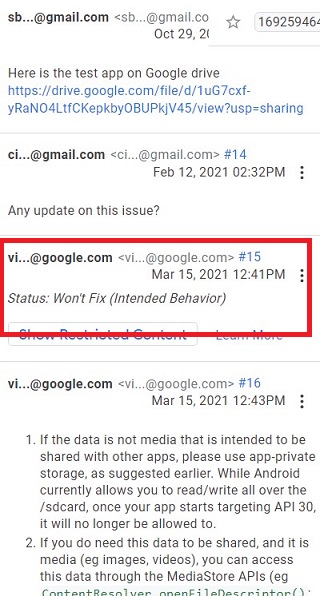The image displays a detailed email thread involving user interactions with Google Drive through Gmail. The email thread begins with a message from "SBA Gmail" dated October 29th (year obscured), which includes a series of numerical identifiers such as "169, 259," situated to the right where you can also favorite the message.

The initial email's subject states, "Here's a test app for Google Drive," followed by a blue hyperlink, indicating a clickable link. Beneath this, there’s a response from "CIA Gmail" dated February 12th at 2:32 PM. Next to this timestamp, a dotted icon appears, likely offering options to delete or modify the email.

Further down is a new message with the query, "Any update on this issue?" marked in a conspicuous red box dated March 15th, 2021, at 12:41 PM. The box contains "VI...@Google" with the status indicating "Won't fix (intended behavior)," followed by another blue hyperlink "Show restricted content" with a "Learn more" option beside it.

The thread continues with a response from "VI...@Google.com" on March 15th, 2021, at 12:43 PM, indicating it is the 16th email in the series noted by "hashtag 16" in blue. The email advises:
1. If the data is not media intended to be shared with other apps, use app private storage.
2. If the data does not need to be shared as media, access it via the media store API.

The email content is set against a white background with blue highlights for hyperlinks and numbered responses, and a red background for the crucial status update box.